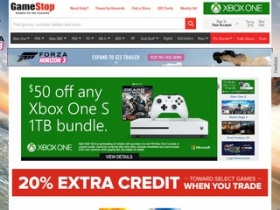This image is a compact screenshot of GameStop’s website. The snapshot is of a small rectangular segment, featuring the iconic GameStop logo at the top left. The logo displays 'Game' in bold black letters and 'Stop' in bold red letters, set against a clean, white rectangular background. To the right of the GameStop logo, there are five small red buttons aligned horizontally. Towards the far right of the top row, there is an Xbox One logo on a dark green background, with 'Xbox One' displayed in white text alongside a white Xbox emblem.

Beneath this top row, the second row contains a search bar centered on a white rectangular background, accompanied by a red square button for initiating searches. Adjacent to the search bar are a cart button and two smaller buttons, presented in light gray text boxes.

Further down, there is a notable long black rectangle, serving as a navigational bar, with a shorter red rectangle positioned on its right end, containing small clickable buttons. Below this navigation bar, the website displays several advertisements, including a prominent dark green ad promoting a $50 discount on an Xbox One S bundle.